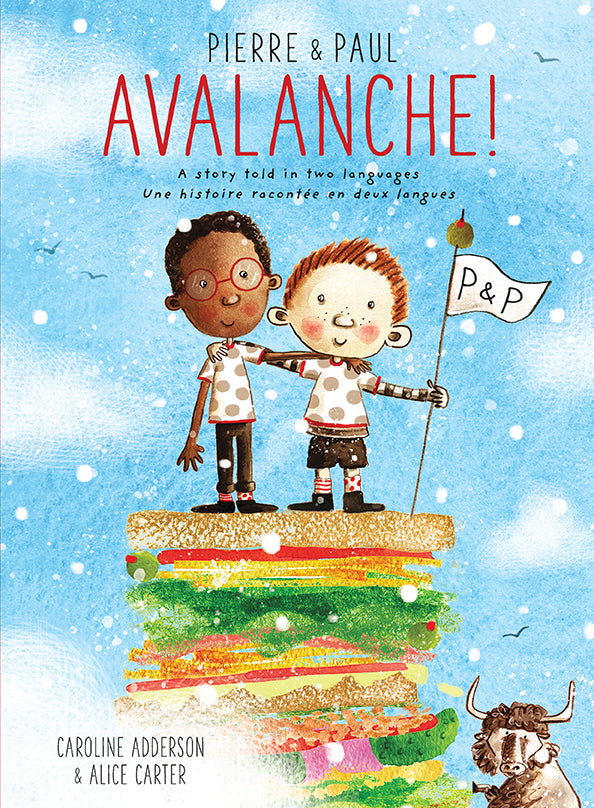This cartoon-style drawing, featured on the cover of a children's book titled "Pierre and Paul Avalanche," is set outdoors under a sky filled with clouds, snowflakes, and little birds. The main background is a serene sky blue. Dominating the scene are two young boys, one black and one white, standing side by side atop a gigantic, multi-layered sandwich filled with appetizing details such as layers of bread, lettuce, tomatoes, cheese, yellow onions, pickles, meat, and more.

The black boy, positioned on the left, is wearing red glasses, a white t-shirt with light brown polka dots, long black pants, black shoes, and red socks—one striped, the other with polka dots. His hair is short and curly brown. The white boy on the right sports short red hair, a matching white t-shirt with light brown polka dots, black shorts, and red socks—one striped and the other with polka dots. He holds a flagpole topped with an olive and a banner that reads "PNP." Both boys are smiling and have their hands on each other's shoulders, symbolizing friendship.

The bottom right corner features a small but determined bull with two horns, seemingly trying to climb the towering sandwich. In the bottom left, the authors' names—Caroline Adderson and Alice Carter—are prominently displayed. The title "Pierre and Paul Avalanche" appears at the top in bold letters, with the phrase "A story told in two languages" and its French translation, "Une histoire racontée en deux langues," just below it.